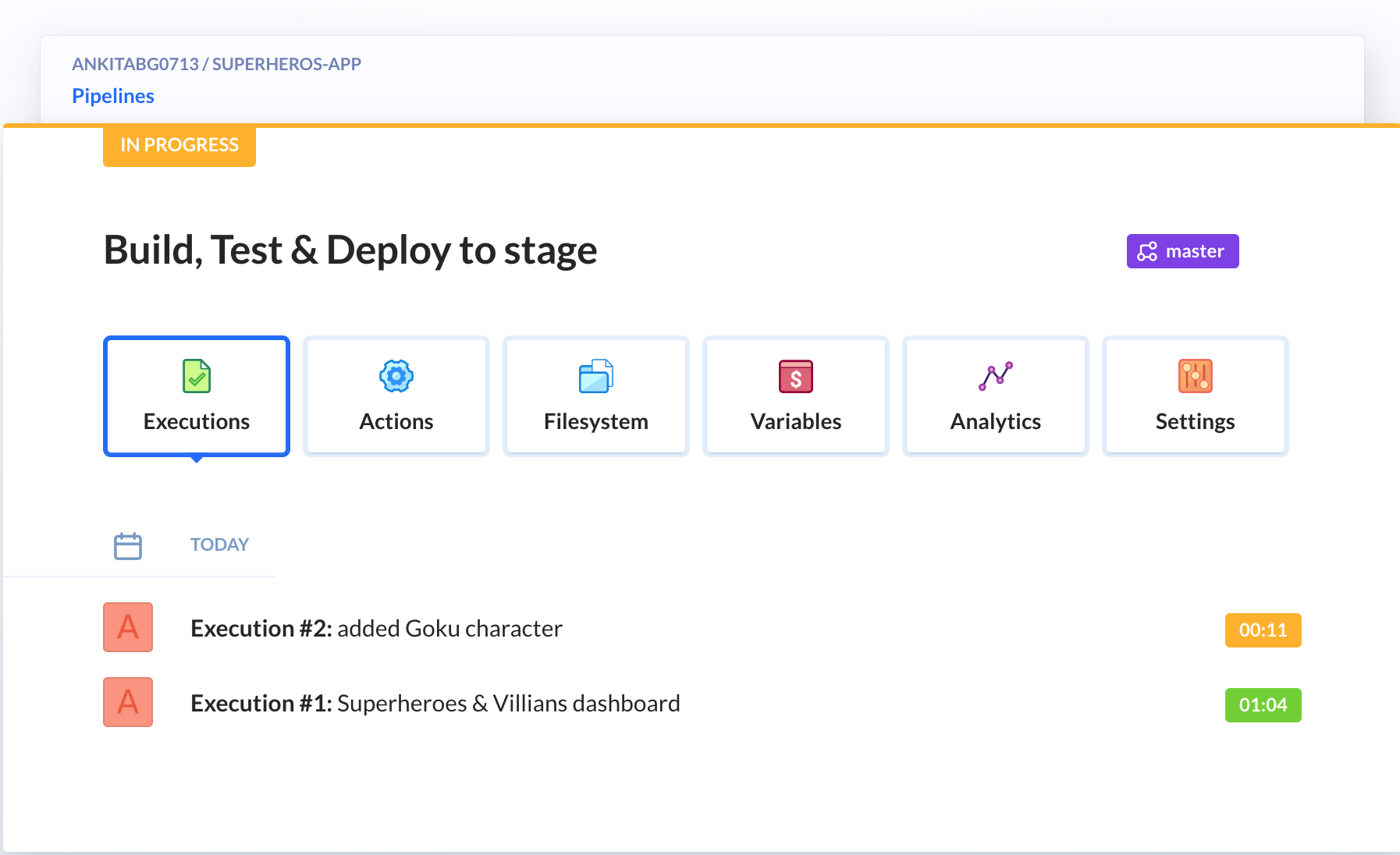**Screenshot Description from GitHub Repository**

The screenshot displays a segment of a GitHub repository, specifically from the path `Go 7/13/superheroes.app`. 

At the top, there is a prominent blue header labeled "Pipelines" with an associated orange indicator stating "In Progress." Below this, a series of pipeline stages are listed: "Build, Test, and Deploy to Stage." 

Towards the right, a purple box with the label "master" signifies the current branch.

In the next row, there is a blue box labeled "Executions," indicating the current active process. Alongside this are additional section headers: "Actions," "File System," "Variables," "Analytics," and "Settings."

Underneath is a timestamp showing "Today," followed by a series of execution logs. The first log entry features a red box with a capital "A" and reads "Execution number 2: Added Goku character," next to which there is an orange box denoting "11 seconds" as the duration for this execution.

The following log entry shows another red box with an "A" depicting a task labeled "Superheroes and Villains Dashboard" which took "1 minute and 4 seconds" to complete.

These logs and timestamps suggest active development work, likely on a game project involving superhero characters.